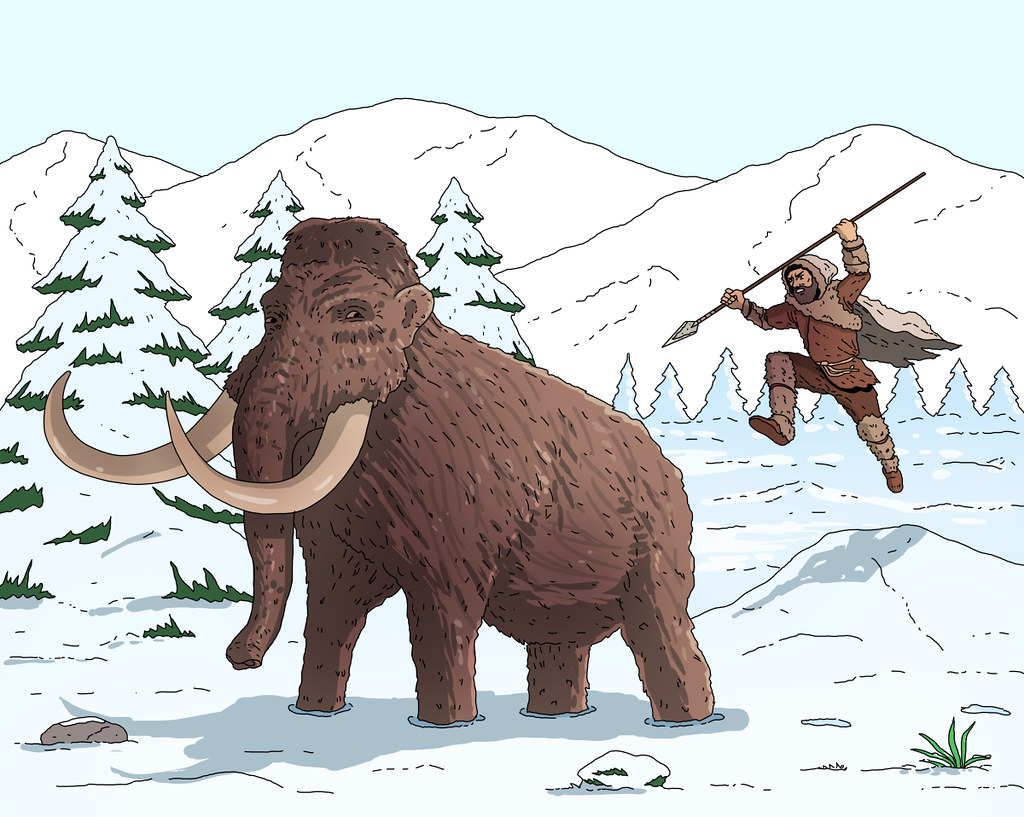In this detailed pen and ink and wash illustration, an artist vividly captures a hunter from days past, mid-leap with a long spear, aiming at a majestic woolly mammoth. The mammoth, with its long, curved tusks and small ears, stands incredulously amidst a snowy landscape, glancing backward at the approaching threat. The hunter, rugged and bearded, is dressed in a homemade ensemble of furs, including knee-high boots, gaiters, a hood, and a cape. He lunges from a snow-covered hill, poised to strike. The background features snow-capped mountains under a faint light blue sky, with snow-covered evergreen trees, some with hints of green trim, and rocks scattered throughout. Small patches of greenery peek through the snow, adding subtle details to this prehistoric winter scene.